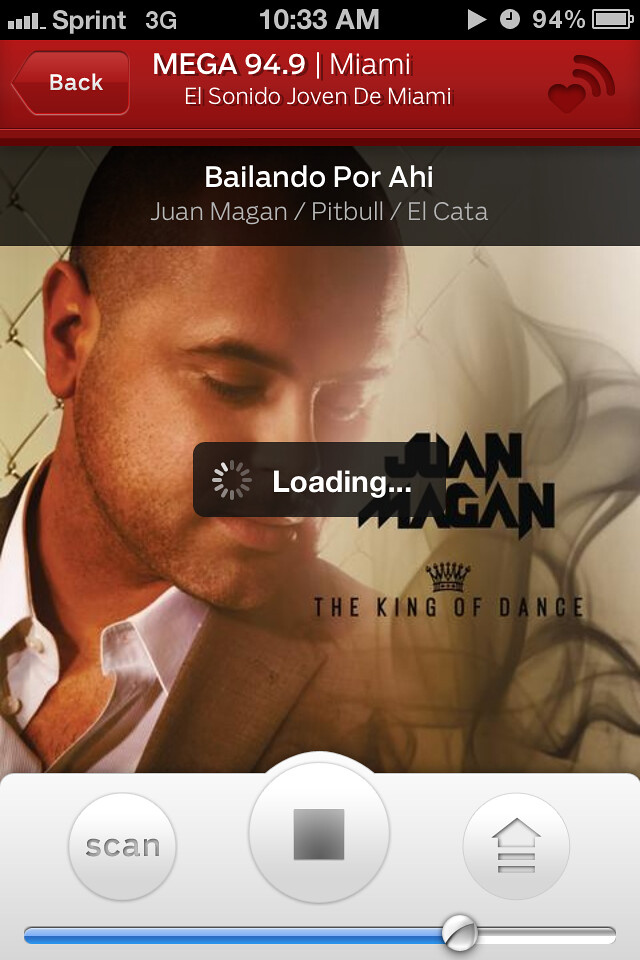The screenshot captures an old iPhone or iPod screen displaying a music app interface under the Sprint 3G network at 10:33 AM with a battery charge of 94%. At the very top, a black bar shows the status icons, including signal strength, time, and battery percentage. Below that, a red section features a "Back" button, with "Mega 94.9 Miami, El Sondito Joven Del Mari" centered next to a heart icon. In the main viewing area, a gray rectangle with white text saying "loading..." overlaps a circular icon with spinning lines, indicating a loading process. The background image is of a man with stubble, eyes closed, a white light reflecting off the right side of his face, wearing a brown suit and an unbuttoned white shirt. Overlaying this image is black text that reads "Juan Megan / Pitbull / Ilocata" and "Valadano Por Ahi," with a subtitle, "The King of Dance," and a small crown icon beneath it. At the bottom, a light silver section contains three circular icons: "Scan" on the left, a central gray square, and an upward arrow on the right. A blue bar with a slider, positioned around 75%, runs along the bottom, indicating playback progress.